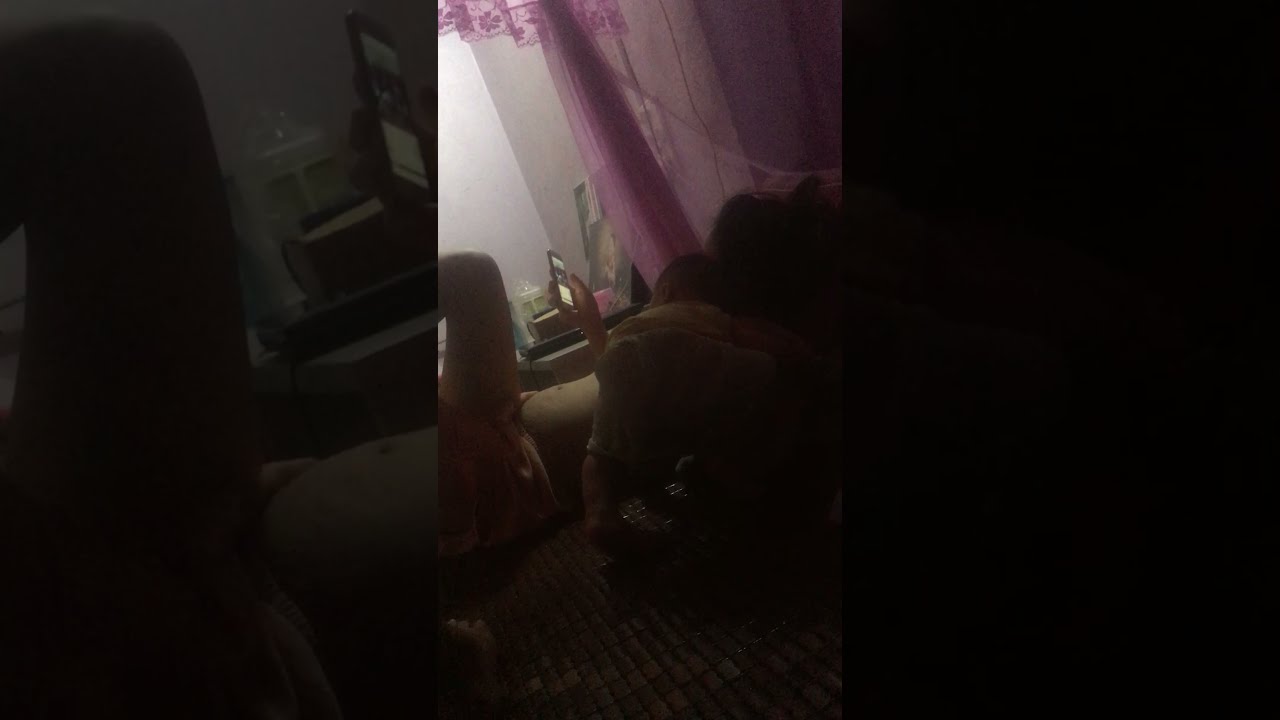In this image, dimly lit and hard to discern at first glance, a serene scene unfolds. Central to the composition is a person lying on their back on a mat or bed, their right arm propped up while they hold a cell phone, seemingly engrossed in a video. Beside them, a small child rests closely, likely nestled on the person's chest or side, also peering at the screen. The child’s position suggests they are partially atop the adult, with one knee bent and the other foot resting on the mat.

Adding to the intimate ambiance is a draped, pinkish-purple silk or lace curtain hanging from the upper right, partially enclosing the sleeping area and contributing to the cozy, private setting. The mat itself appears to have a brown, tiled pattern. The background reveals faint details of a bedside table or surface, adorned with photos and miscellaneous items, illuminated by an unseen light source that brightens the edge of the adult’s belly. Further back, the dimly visible white walls and paintings leaning vertically add depth to the image.

Despite the deep shadows dominating the scene, the gentle light and soft textiles create a comforting and warm environment, capturing a tender moment between the adult and the child.